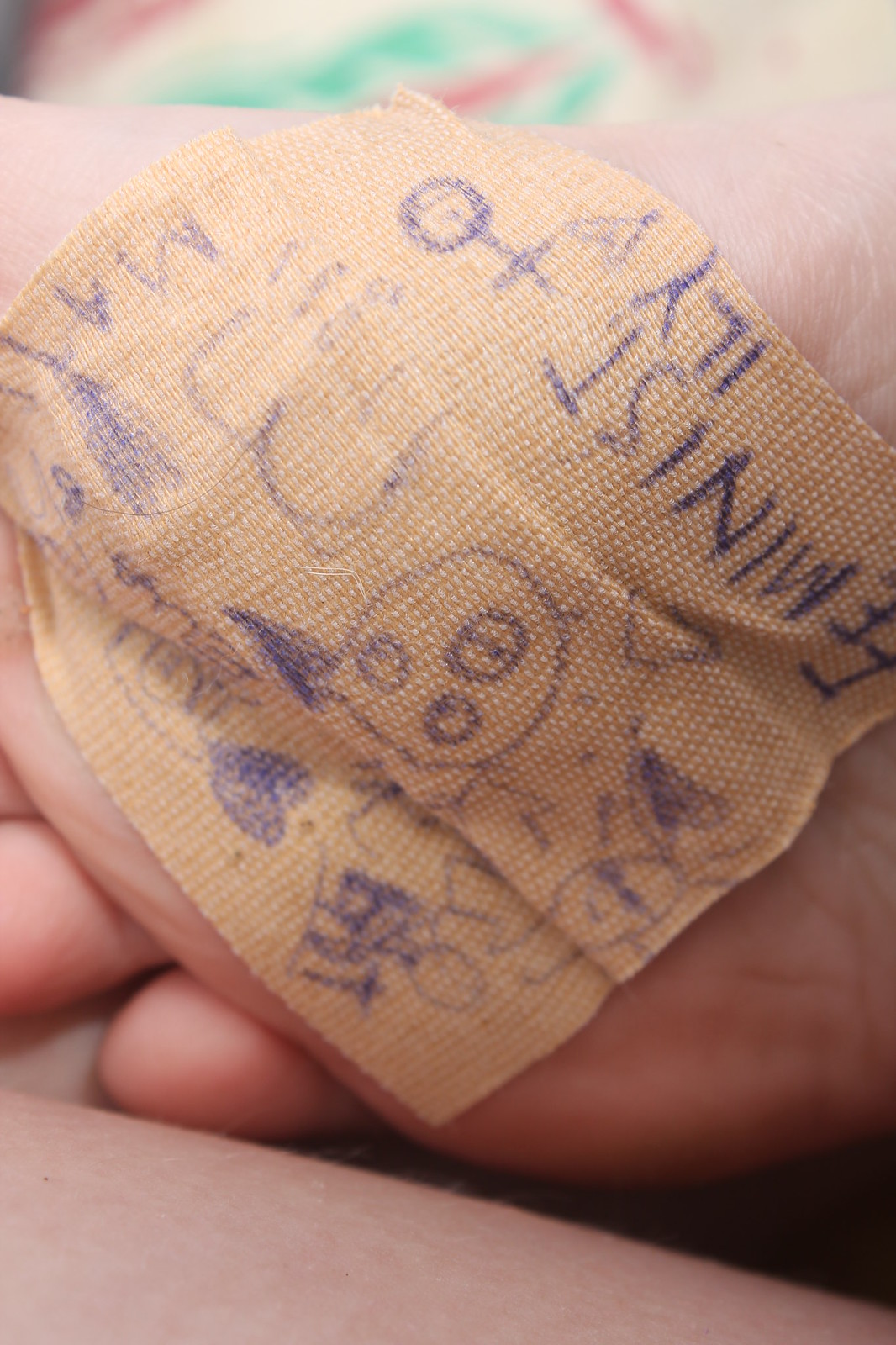This photograph captures a close-up of a small foot, likely of a baby or young child, oriented upside down with toes visible at the top of the image. The foot rests on another part of the body, possibly a leg, seen in the bottom left corner of the photo. Covering the ball of the foot is a large square bandage, reminiscent of a band-aid. The bandage features various scribbles and doodles drawn with a blue pen. Among the drawings are a stick figure with a round head, a heart symbol, and a face with large circular eyes and a round mouth. Upside down text on the bandage reads "FEMINIST" next to the female symbol (circle and plus sign), as well as "ILY" (I Love You). The overall scene suggests a personalized, caring gesture with playful, graffiti-like art added to the bandage.